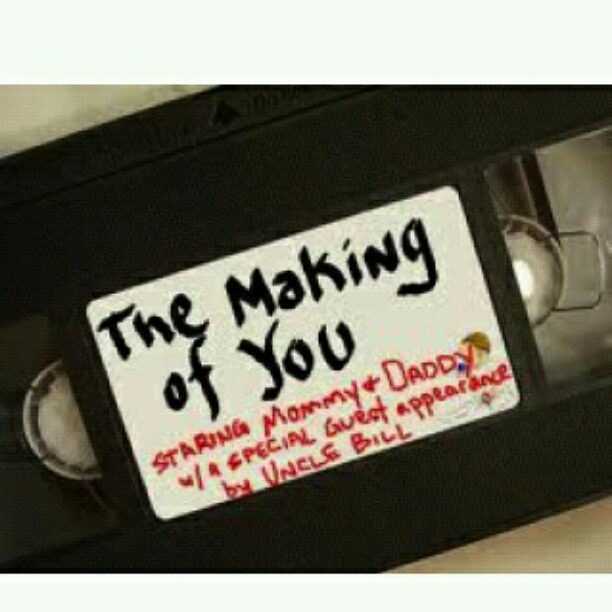The image is a square photograph featuring a black VHS cassette tape, partially cropped at the top, left, and bottom-right edges. The photograph appears slightly pixelated and low in quality. The tape is positioned against an off-white, tan-colored surface. At the top and bottom of the image are thin, light greenish-blue rectangles that frame the image.

Centered on the cassette is a white rectangular label with curved corners. The label's text is primarily in black font, reading "The Making of You," while the bottom portion features red handwriting that says, "Starring Mommy and Daddy with a special guest appearance by Uncle Bill." On the left side of the cassette, a full spool of film is visible through a clear viewport, indicating that the tape is fully rewound and ready to play from the beginning. The right side of the cassette shows an empty spool and a plastic portion that includes a light inside. The overall impression is one of a nostalgic, possibly digitally altered image meant to evoke memories or convey a sentimental message.